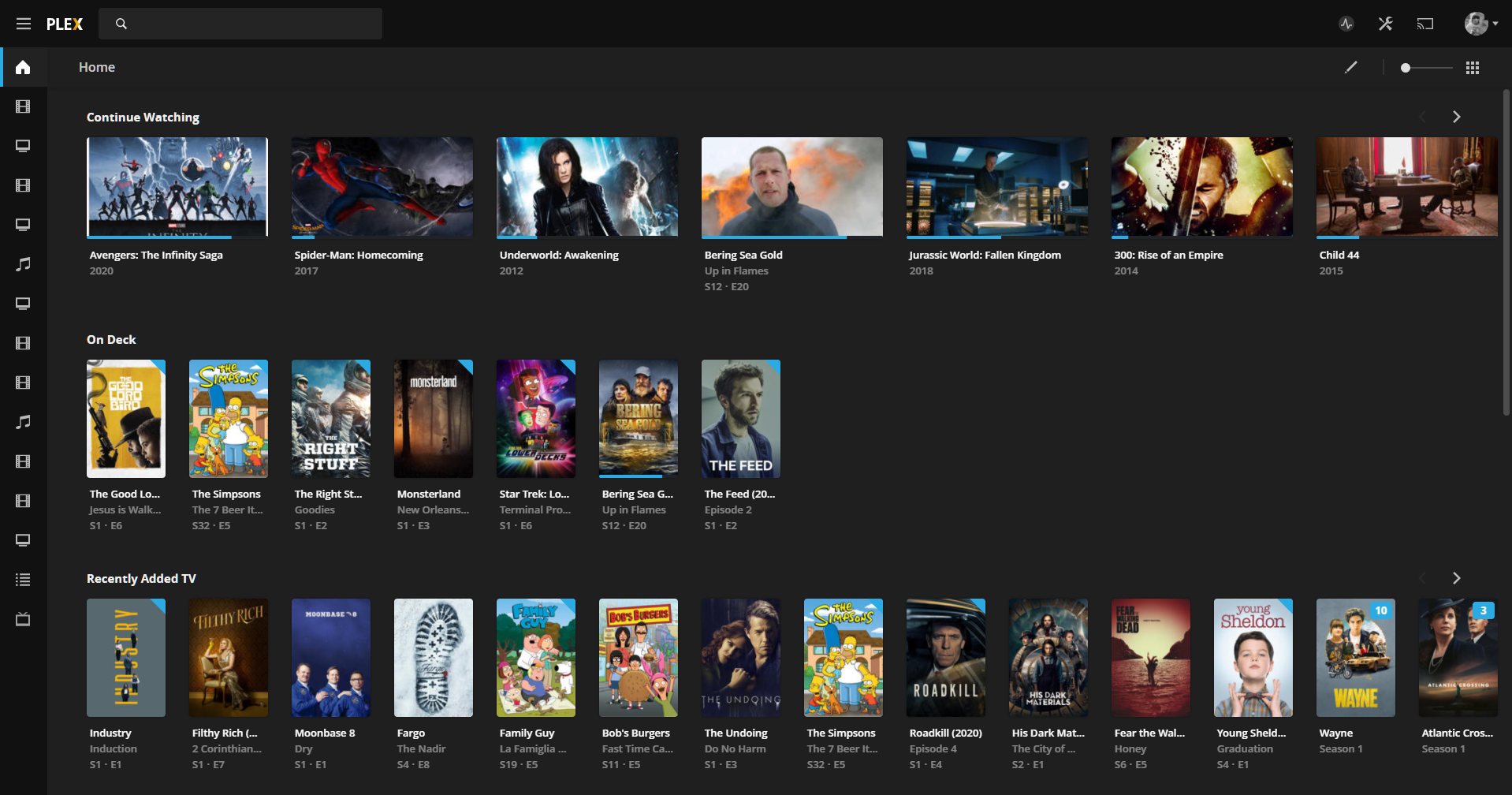This image showcases the desktop version of the Plex user interface as viewed on a personal computer or laptop, which differs from its TV interface. Plex, a platform similar to Netflix but initially focused on allowing users to download and stream movies through their social media devices, has since evolved into a free streaming service, akin to Tubi, Freevee, and Pluto TV.

The screen exhibits several sections of the Plex webpage. The "Continue Watching" section appears first, displaying a collection of movies that the user hasn’t finished watching. This is followed by a list of saved movies, either bookmarked by the user or recommended by Plex's algorithms. The final section shown is "Recently Added TV," featuring a mix of well-known and lesser-known television shows. Though the titles are somewhat indistinct, they hint at the wide variety of content available on the platform. 

Overall, this detailed view highlights Plex's robust interface and its capability to go beyond just streaming downloaded content, offering a comprehensive entertainment service on par with other free streaming platforms.